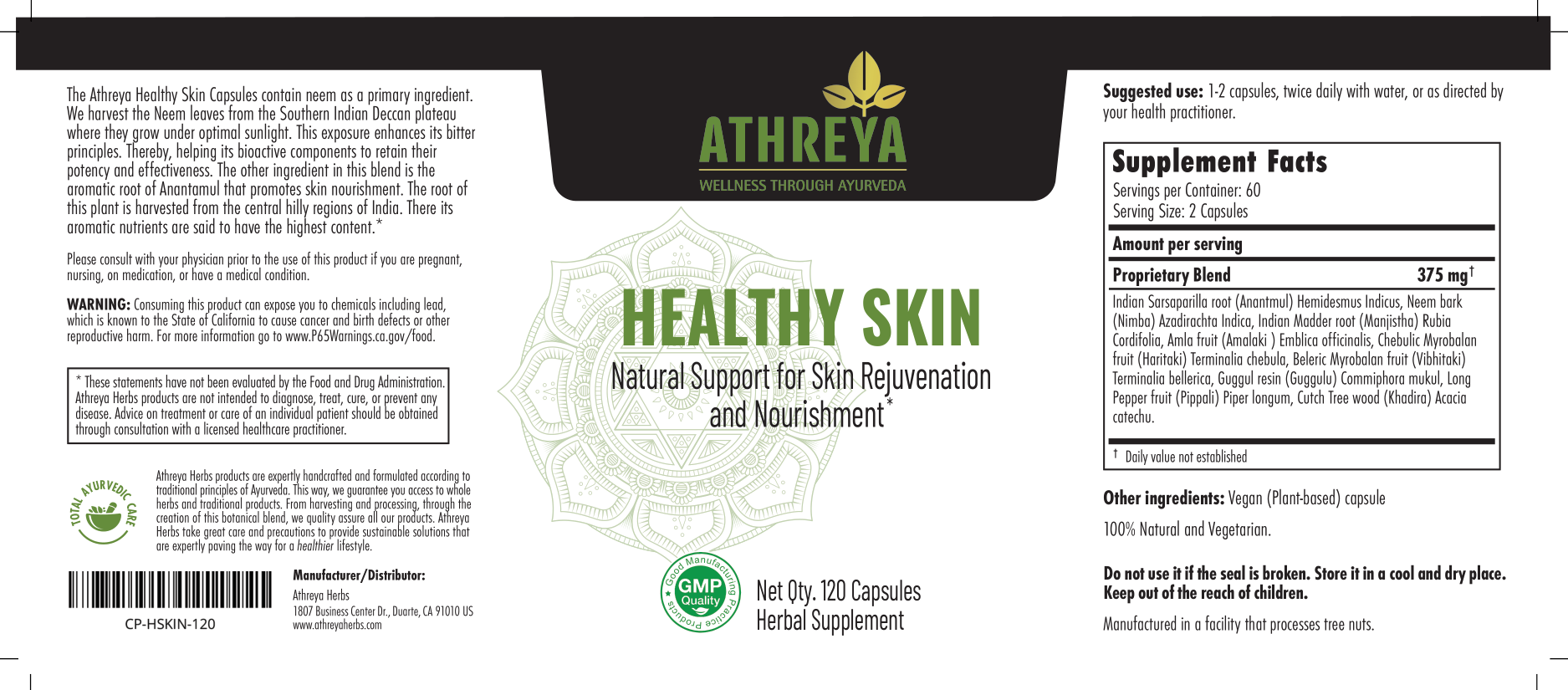The image is a digital screenshot of a product label for a supplement bottle, characterized by a black border at the top and a primarily white background below. The black band at the top features a green logo of three leaves sprouting from the letter 'Y', along with the brand name "ATHREYA" (A-T-H-R-E-Y-A) in green text. Below this, a smaller green text reads "Wellness through Ayurveda" on a yellowish line. Prominently, the label contains large green text stating "Healthy Skin", followed by smaller black text that reads "Natural Support for Skin Rejuvenation and Nourishment".

On the left section of the label, there is a detailed product description and a warning label, with a UPC symbol at the bottom. The center part of the label, considered the front, has a GMP quality certification logo, and next to it, it states "Net Quantity: 120 capsules herbal supplement". A green mandala design is faintly visible in the background. 

The right side lists the suggested use instructions, advising one to two capsules twice daily with water or as directed by a health practitioner. It also includes supplement facts in a bordered box, along with ingredients, which are 100% natural, vegan, and vegetarian. Additional cautionary statements are noted, such as "Do not use if the seal is broken," "Store in a cool and dry place," and "Keep out of the reach of children." It also mentions that the product is manufactured in a facility that processes tree nuts. There are crop marks at all corners of the label, indicating it is ready for printing.